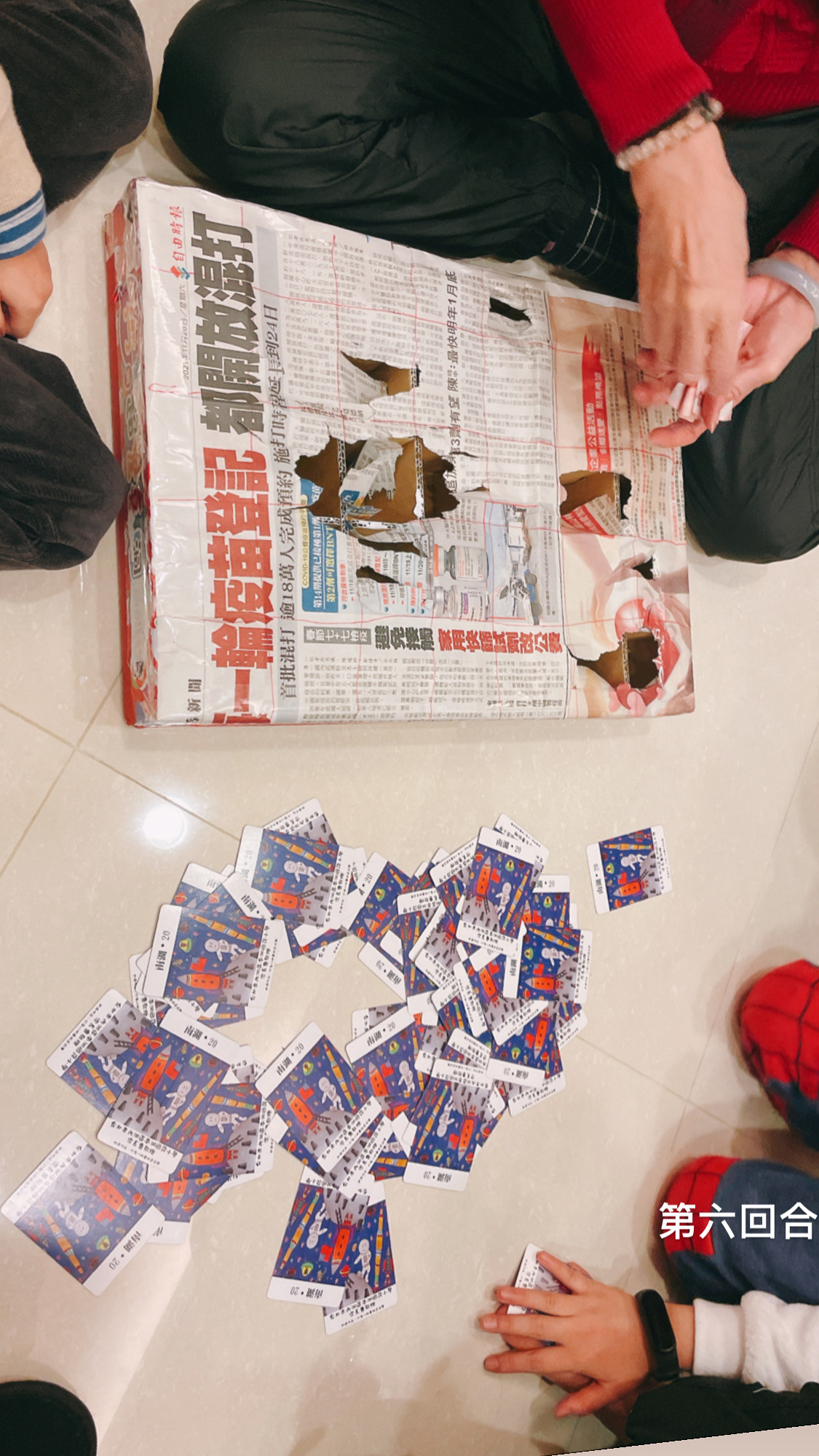A rectangular photograph captures an engaging scene of four individuals absorbed in a lively card game. The composition features each player positioned in one of the four corners of the image, viewable predominantly from the waist down to their hands. Each participant emanates a unique sense of style and age. In the bottom left corner, a younger person is dressed in gray denim pants and a long-sleeve white shirt, accented with blue and white stripes at the cuff. Contrastingly, the person in the top right corner, also younger, sports black pants paired with a vibrant red long-sleeve shirt and adorns their wrist with a beaded bracelet and a white plastic bracelet. The top left corner reveals an older individual, although much of their attire is not detailed in the caption, and the bottom right corner shows only a foot. Scattered across the game area are numerous cards, each featuring a vivid illustration of an astronaut beside a rocket ship, suggesting an intriguing space-themed card game. The intimate framing and details of the players' clothing and accessories evoke a sense of camaraderie and shared focus within this moment of leisure.